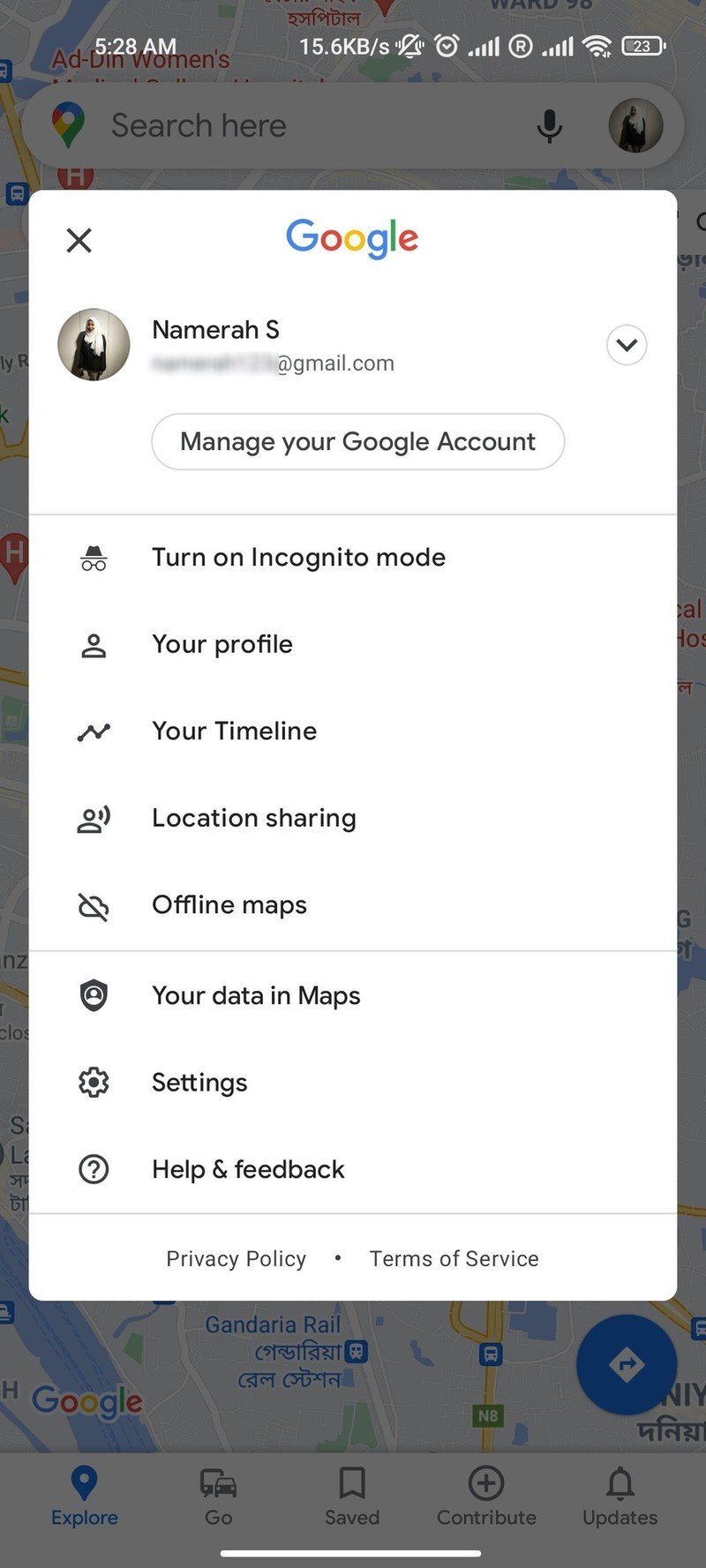This image is a screenshot taken from a smartphone, displaying a multi-layered interface. The primary screen features a grayed out, opaque background that partially obscures an underlying application, in this case, a map, though the specifics of the map are not visible. 

In the top-left corner of the screen, a status bar is visible, showing the time as "5:28 AM" and data transfer rate as "15.6 KB/s". The icons present include a crossed-out alarm clock, a standard alarm clock symbol, two service bars indicating signal strength, a Wi-Fi icon, and a battery icon showing a 23% charge.

Overlaid on this background is a detailed Google account management pop-up. This window has a familiar Google branding with an "X" button for closing it in the top-left corner. At the center is the Google logo, followed by the partial, blurred email address of the user, "Nomera S," and a user profile picture to the left. To the right of the email address is a drop-down menu. Beneath these elements is a button labeled "Manage your Google Account."

Further down, a list of options is presented in a vertical layout which includes:
- Turn on Incognito Mode
- Your Profile
- Your Timeline
- Location Sharing
- Offline Maps
- Your Data in Maps
- Settings
- Help and Feedback

At the very bottom of the pop-up, there are links to Google's "Privacy Policy" and "Terms of Service."

Despite the overlay, the faintly visible map background indicates an active navigation or map application, suggesting the user might have been in the middle of a search or route planning when this screenshot was captured.